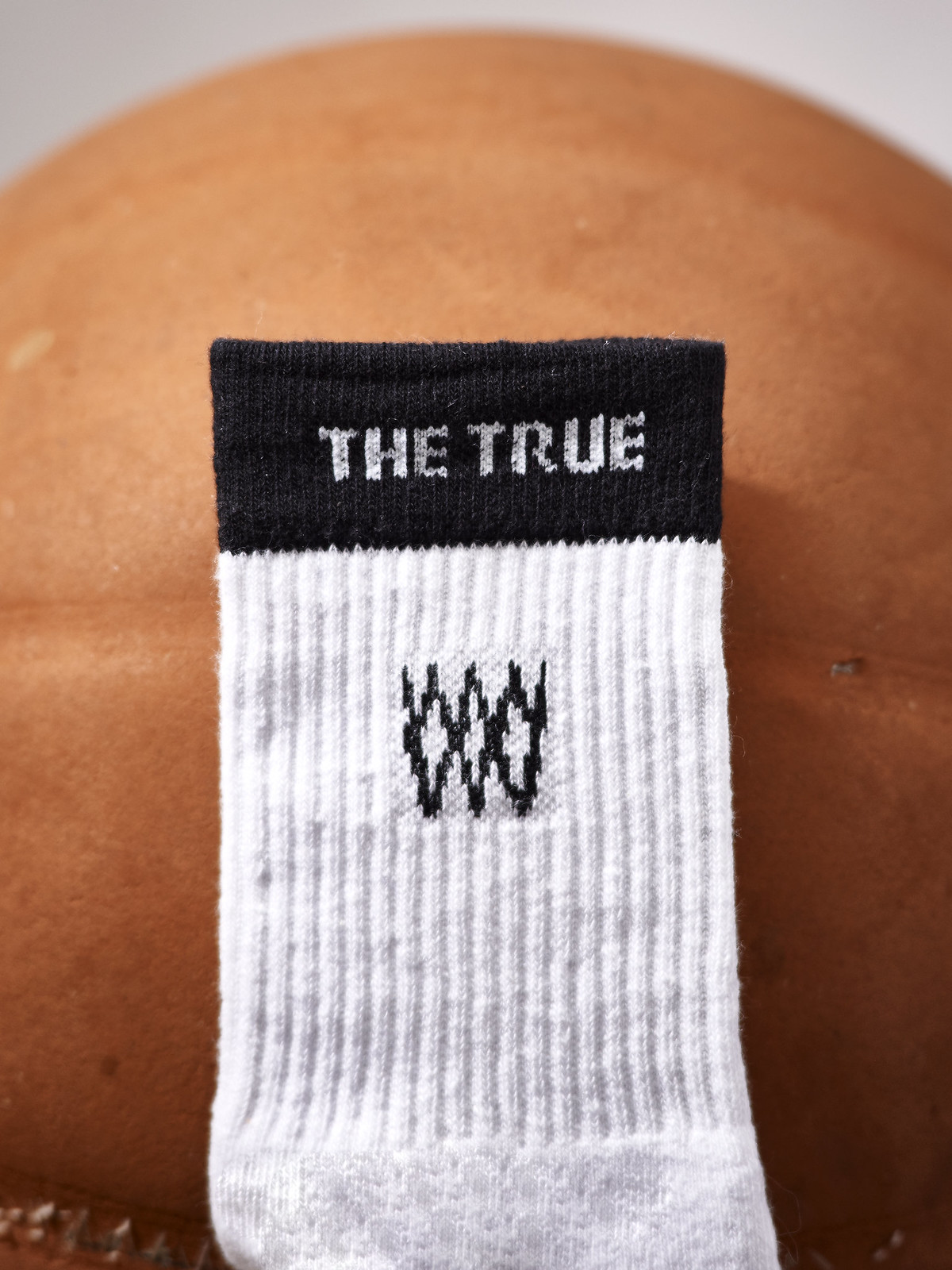The image depicts a white tube sock prominently positioned against an orange, rounded object, possibly resembling a ball or a pumpkin lying on its side. The sock features a black band at its top edge with the white stitched words "the true." Below the band, two overlapping black zigzag patterns, akin to the letter 'W,' are embedded in the fabric, possibly forming a logo. The sock extends the full height of the image but is cut off at the bottom, excluding the heel. The background shows a gray surface in the upper corners, with the orange object's texture featuring small horizontal grooves near where the sock's white fabric begins and near the corners at the bottom of the image.